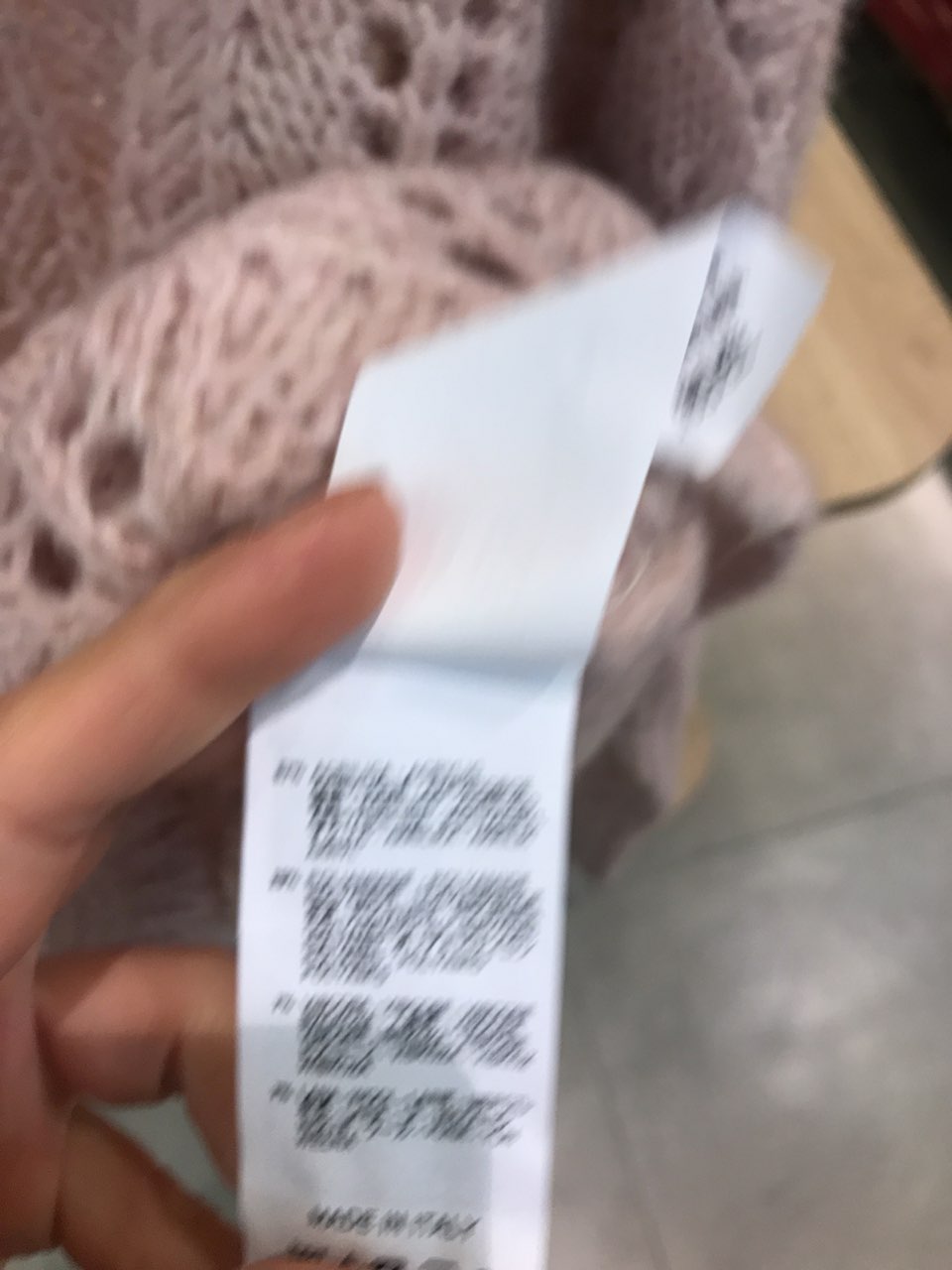The photograph depicts a close-up of a hand holding the internal tag of a knitted garment, which appears to be a light dusty pink sweater. The focus is on two white paper tags attached to the inside seam of the sweater. One tag is flipped up, obscuring any text on its back side, while the visible tag shows a partial and blurred inscription at the bottom, suggesting the origin of manufacture but not clearly indicating the country. The backdrop of the image reveals a tiled tabletop, adding a touch of domesticity to the setting. The hand holding the tag is centrally positioned, emphasizing the details of the tag and the texture of the knitted fabric.